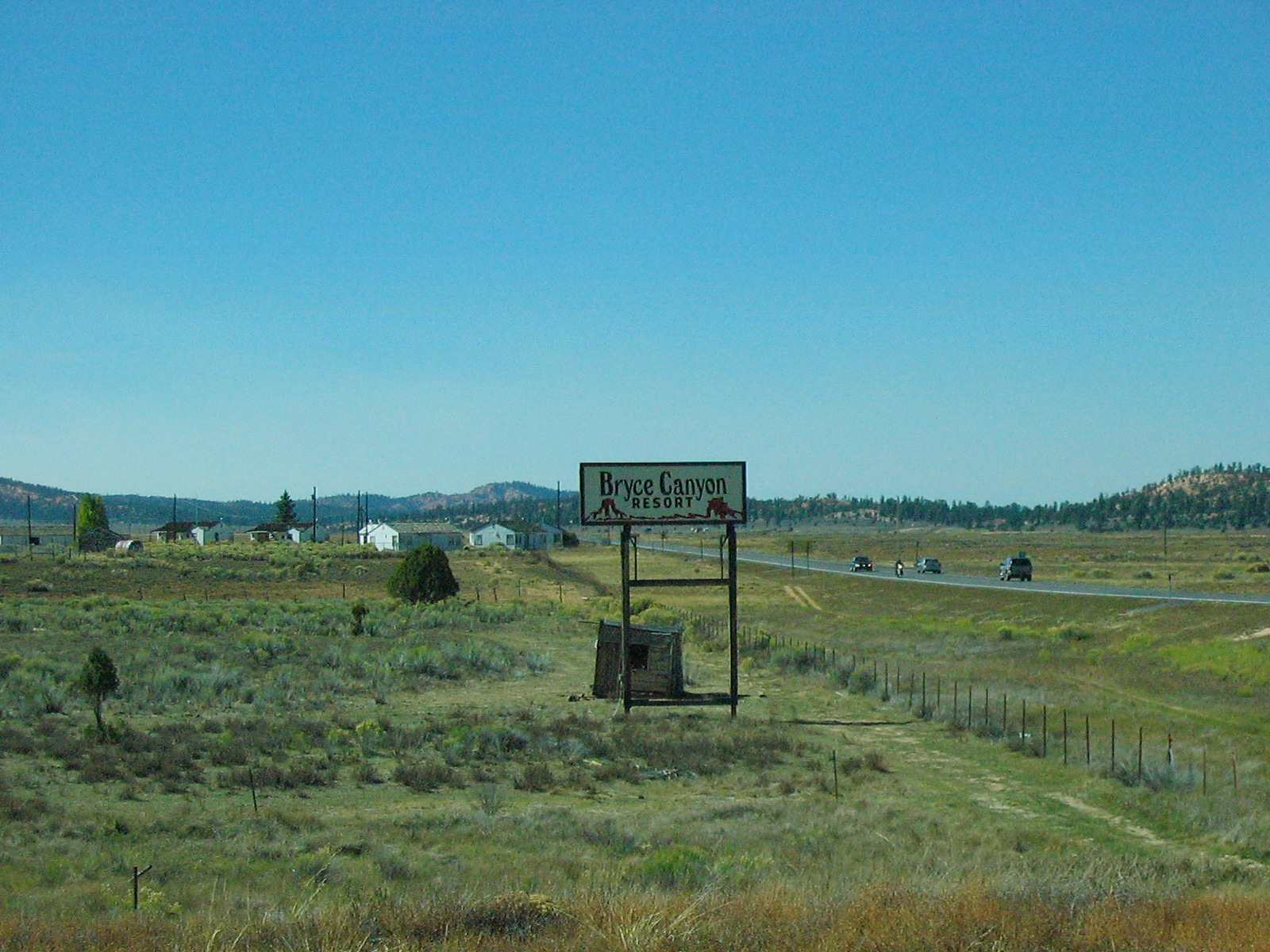The outdoor image captures a scenic view of Bryce Canyon Resort under a clear blue sky. In the foreground, there is a mix of green and dry grass, bordered by numerous fence posts. To the extreme right, a patch of gray ground is visible, accompanied by several green trees. In the background, dark green buildings with sloped roofs and blue wooden panels add a rustic charm to the landscape. Hills covered in dense forests stretch across the horizon, creating a picturesque backdrop. Prominently displayed is a white sign on the right that reads "Bryce Canyon Resort." The entire scene is framed by mountains on both sides, enhancing the natural beauty of the resort.